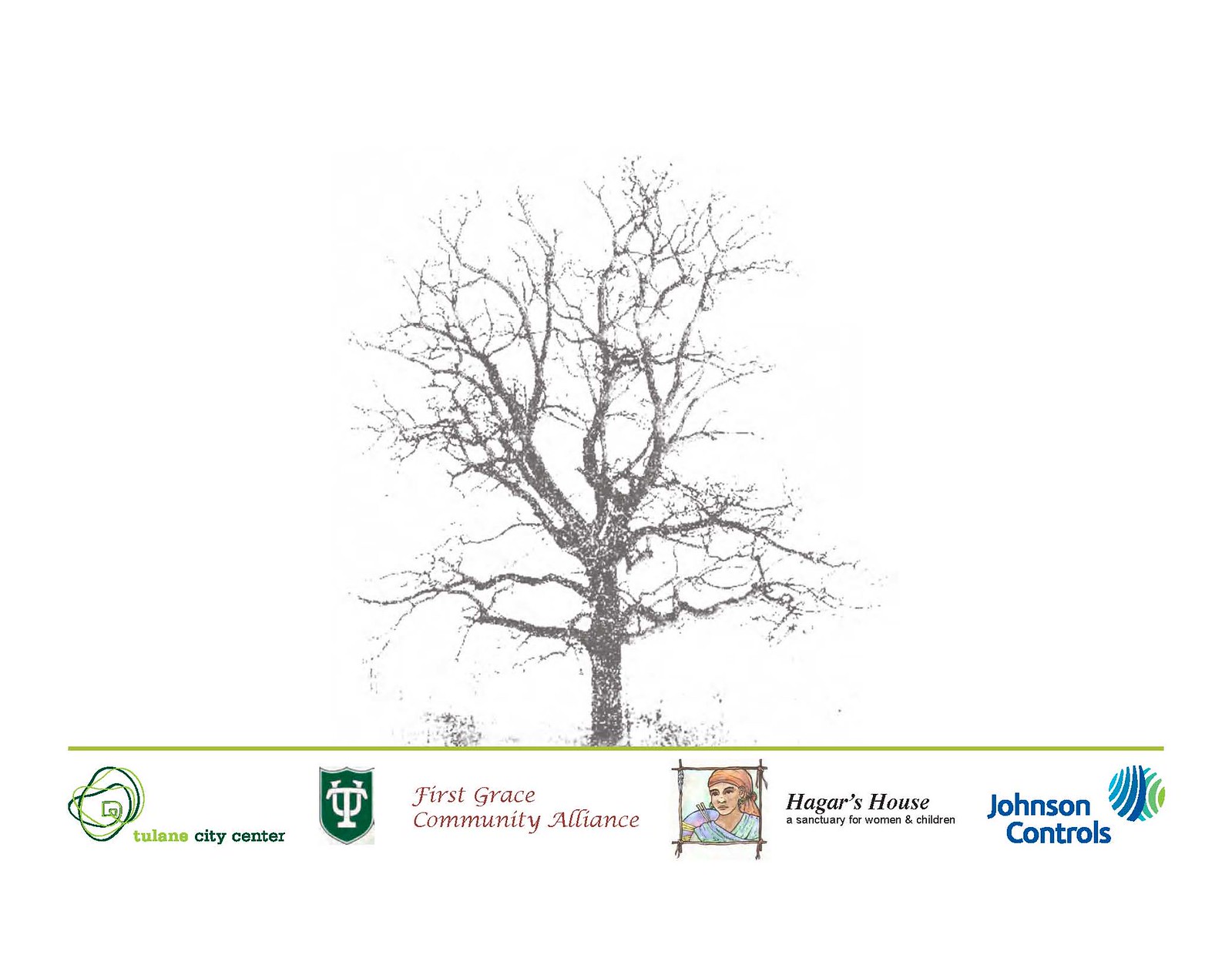The image features a stark winter scene of a barren tree, its dark, leafless branches extending approximately three stories high, against a plain white background. A yellow line runs horizontally across the bottom of the image, beneath which the background remains white. Below this line, there are four advertisements: 

1. **Tulane City Center**: Located in the bottom left corner, this advertisement is marked by the words "Tulane" in green followed by "city center" in black, accompanied by an emblem in black and green.
2. **First Grace Community Alliance**: Next to the first advertisement, a black shield with "UT" in white lettering sits beside the name "First Grace Community Alliance" written in a reddish hue.
3. **Hagar's House**: This advertisement features a symbol resembling four intersecting sticks or arrows and an image of a woman with reddish-blonde hair, wearing a blue shirt and carrying a blue item on her back. The words "Hagar's House: A Sanctuary for Women and Children" are written in black.
4. **Johnson Controls**: The final advertisement to the right showcases the text "Johnson Controls" in blue, next to a blue, green, and yellow circular emblem.

This detailed depiction encompasses the barren tree at the top and the series of advertisements at the bottom, blending both visual and textual elements seamlessly.